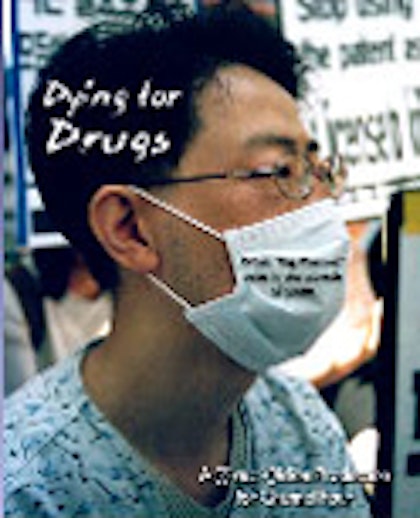The image depicts an Asian man with short black hair and glasses, wearing a light blue top, possibly a hospital gown or scrubs, and a surgical face mask. He is shown in a side profile, looking to the right of the frame, while his face is positioned centrally within the image. The photo is of low quality and appears somewhat blurry, making some details difficult to discern. Written in white text on the side of his head are the words "dying for drugs." Additionally, there is some indiscernible black text on his mask and more blurry text across his chest. Behind him are some signs that are not clearly readable, along with possible shelving, contributing to an unclear background. The overall setting suggests the image might be a still from a TV show or a low-resolution magazine print. The predominant colors in the image include white, black, brown, tan, and blue.